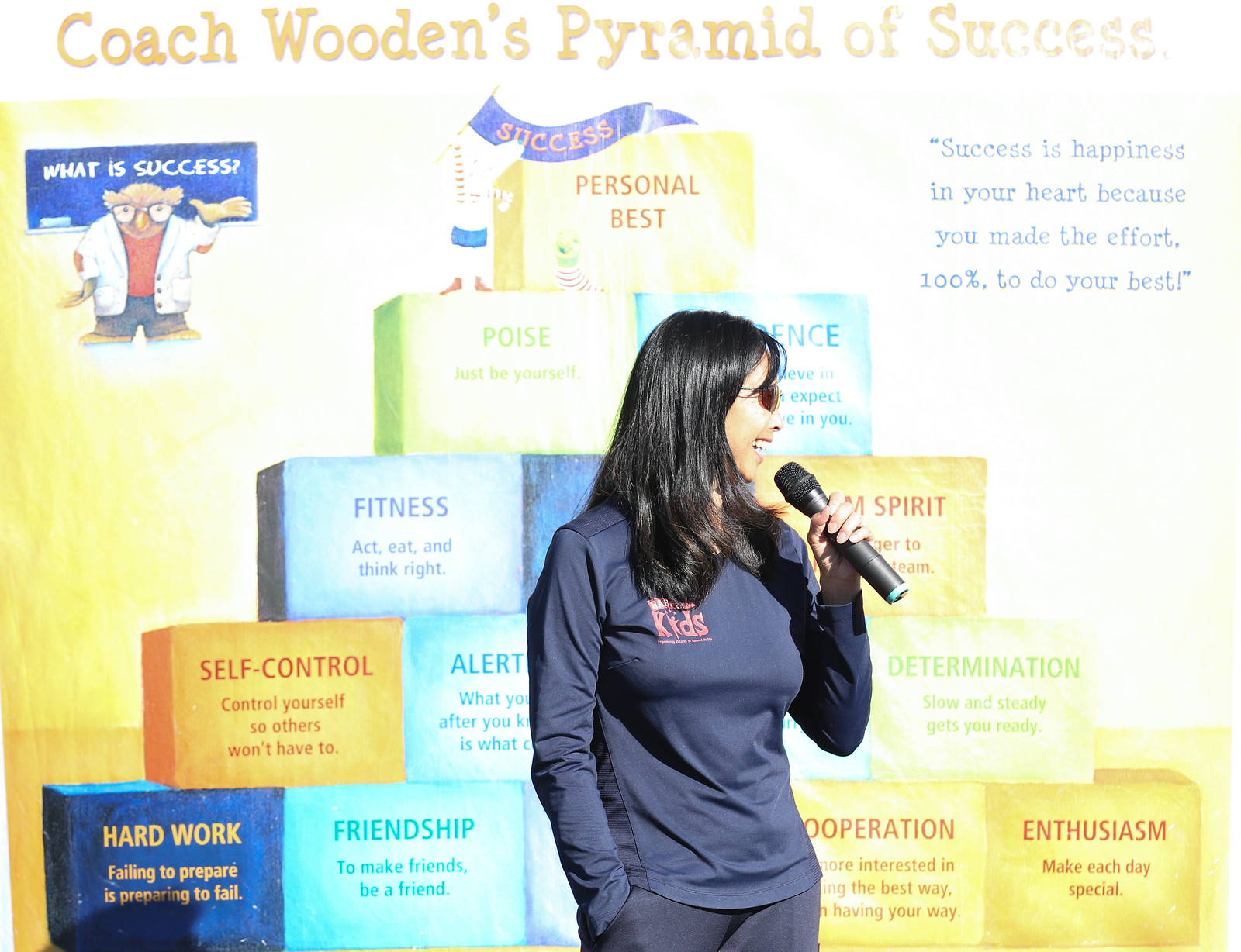In this image, a woman of East Asian descent stands confidently with a microphone in her left hand. She has long, dark hair cascading over her shoulders, and she is dressed in a dark blue, long-sleeved blouse featuring a pink insignia that spells out "K-I-D-S," paired with gray pants and sunglasses. She is positioned in front of a large poster or banner labeled "Coach Wooden's Pyramid of Success," which displays a multicolored pyramid of blocks, each representing different attributes for achieving success.

At the top of the pyramid, the block reads "Personal Best," followed by "Poise" and "Confidence" on the next tier. Below them are "Fitness" and "Team Spirit," while the middle layer includes "Self-Control," "Alertness," and "Determination." The bottom tier shows "Hard Work," "Friendship," with "Cooperation" and "Enthusiasm" partially covered by the woman. The phrases and words on the banner provide guidance such as "Poise: Just be yourself,” “Fitness: Act, eat, and think right,” “Self-Control: Control yourself so others don’t have to,” “Hard Work: Failing to prepare is preparing to fail,” “Friendship: Make friends and be a friend,” and “Enthusiasm: Make each day special.” The woman appears to be delivering a speech or lecture, her demeanor radiating happiness and engagement with her audience.